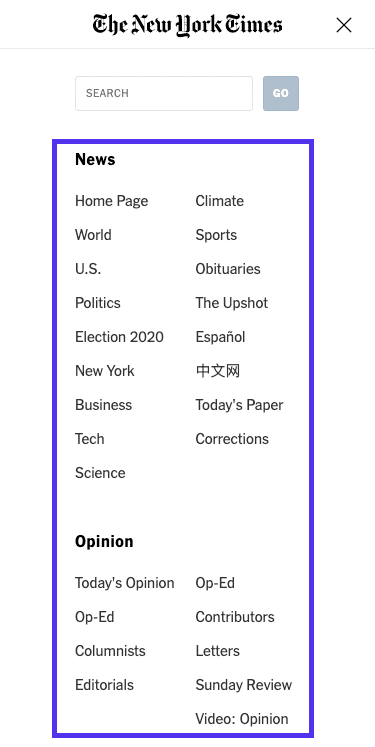This image is a detailed screenshot captured from a cell phone, displaying the New York Times website. At the very top, the familiar “The New York Times” logo is prominently featured in bold black text, with a small 'X' icon situated to the right, likely for closing the window or menu. Directly below this header is a white search box, where gray placeholder text reads "Search," accompanied by a gray "Go" button to initiate the search.

Descending further, an eye-catching bright blue outline frames a segment of black text within the box, which prominently states "News" in bold. Underneath this, a series of categorized links are listed: homepage, climate, world, sports, U.S., obituaries, politics, the upshot, election 2020, Español, New York, business, today's paper, tech, corrections, and science.

Following this comprehensive list, the section transitions into "Opinion," displayed in bold black text. The screenshot effectively captures the essential navigation elements and sections available on the mobile version of the New York Times website, providing a clear overview of its layout and available categories.